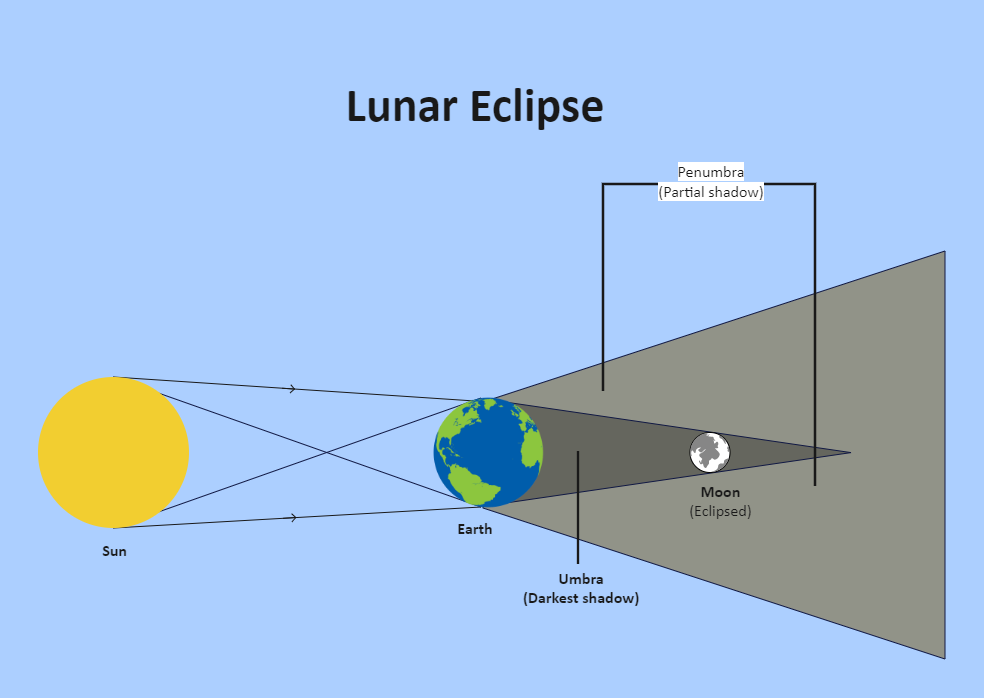The image is a detailed diagram illustrating the process of a lunar eclipse set against a light blue background. The title "Lunar Eclipse" is written in black at the top. On the left side of the image, there is a prominent yellow circle labeled "Sun." In the center of the image, a blue and green sphere labeled "Earth" is depicted. To the right of the Earth, there is a smaller gray and white circle labeled "Moon, Eclipsed."

Arrows extend from the Sun to the Earth, demonstrating the direction of the sunlight. These create distinct triangular shadows between the Earth and the Moon. The smaller, dark gray triangle is labeled "Umbra, Darkest Shadow," showing where the Earth's shadow totally obscures the Moon during an eclipse. Surrounding this, a larger, lighter gray triangle labeled "Penumbra, Partial Shadow" illustrates the area where only a portion of the Sun's light is obstructed by the Earth.

The diagram is a comprehensive visual explanation of how the Earth's shadow causes a lunar eclipse, detailing the spatial relationships and shadow effects of the Sun, Earth, and Moon.